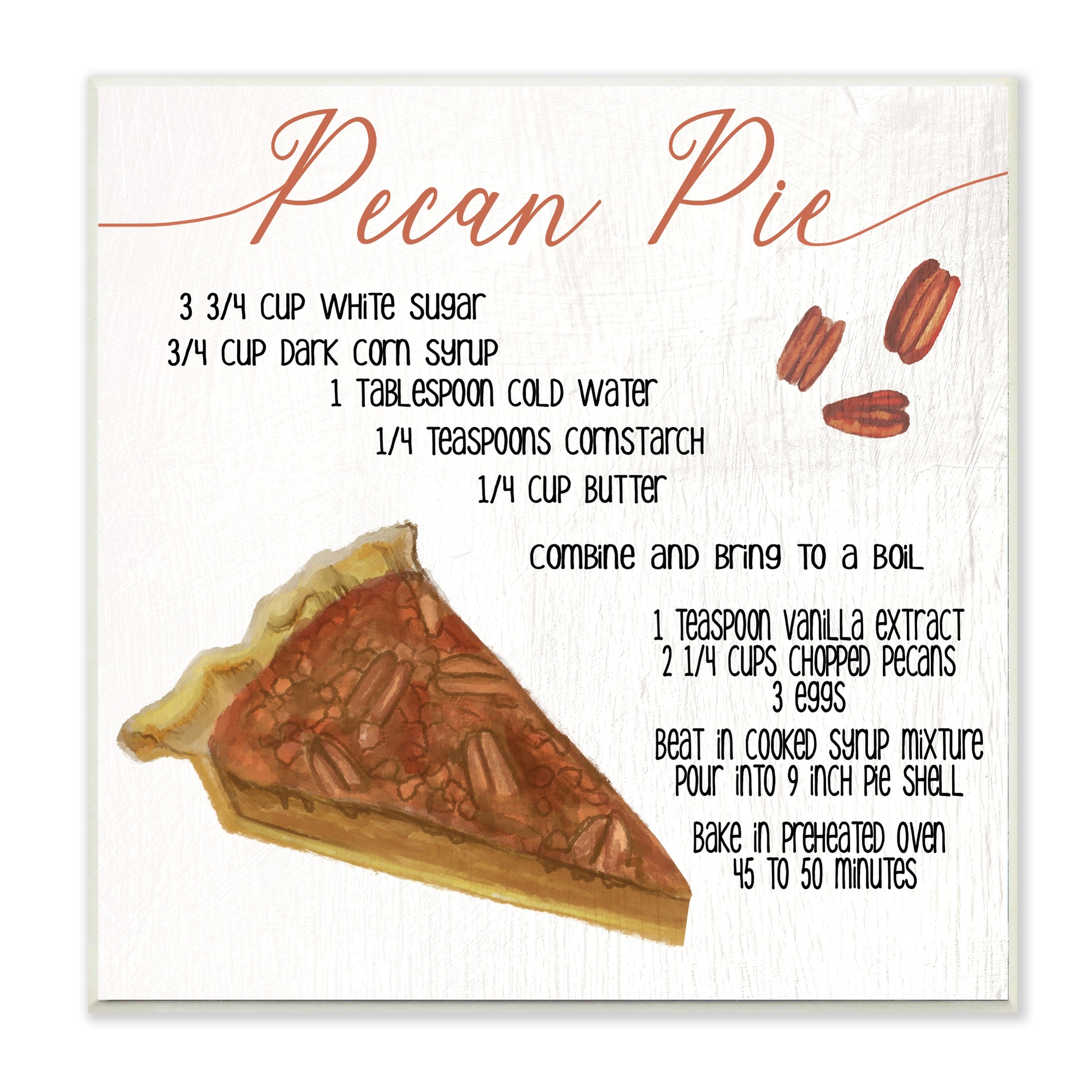The flyer is a square-shaped illustration that appears to be designed like a slightly raised wooden sign. At the top, it prominently features the text "Pecan Pie" in large, light brown script. Below this title, the recipe is listed in all capital letters, running diagonally from the upper left to the bottom right. The recipe details the ingredients and steps: 3/4 cup of white sugar, 3/4 cup of dark corn syrup, 1 tablespoon cold water, 1/4 teaspoon cornstarch, 1/4 cup butter (to be combined and brought to a boil), 1 teaspoon vanilla extract, 2 1/4 cups chopped pecans, and 3 eggs (to be beaten into the cooked syrup mixture). It instructs to pour the mixture into a 9-inch pie shell and bake in a preheated oven for 45 to 50 minutes. To the right of the text, there are small illustrations of brown pecans. On the bottom left, there is a large, triangular slice of pecan pie depicted in a watercolor style, showcasing the beige-colored crust and the brown and cream toppings.